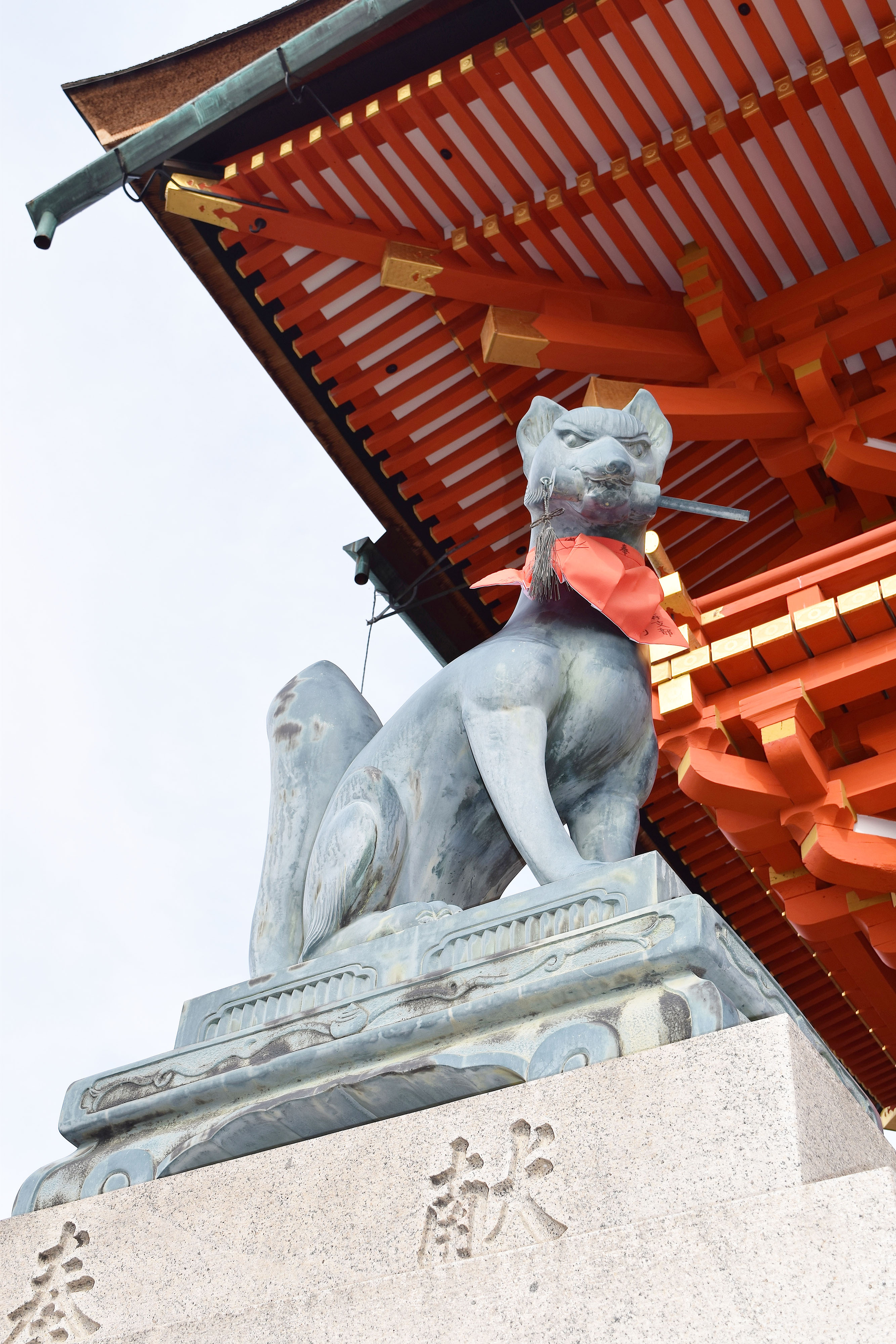This image captures an upward view of a striking and intricate scene. The bottom area features a long rectangular sandstone brick adorned with Asian-style symbols or writing, likely Japanese or Chinese characters. Perched above this is a formidable gray stone statue of an animal, which appears to be larger than a typical cat but smaller than a tiger, resembling both a dog and a cat. The statue has a weathered appearance with black marks throughout its body and it holds an unidentifiable object, possibly a stick, in its mouth. Its eyes convey anger through downward-pointing eyebrows. Above the statue is a roof characterized by a complex array of red beams interspersed with yellow blocks, giving the impression of a traditional Japanese shrine.